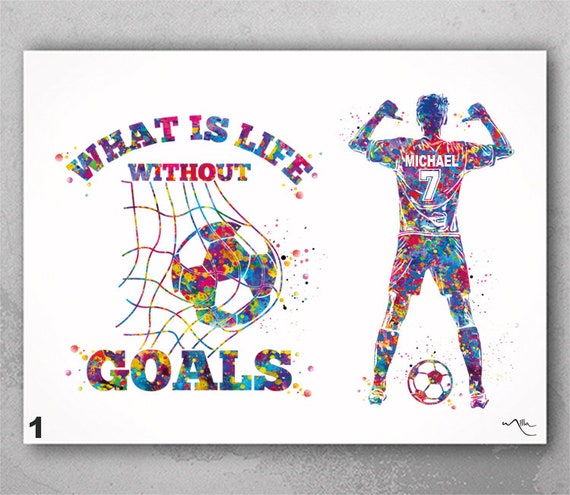The image is a detailed, soccer-themed poster mounted on a textured gray wall. The flat white panel features a prominent number "1" in the lower left corner and is signed "Mila" in the bottom right. The background is predominantly an off-white hue. The central portion of the poster contains arching text that reads, "What is life without goals?" in a colorful, splatter-brush font incorporating shades of blue, yellow, and red within each letter. 

Between the words "without" and "goals," a vibrant depiction of a multicolored soccer ball is shown being kicked into a similarly multicolored mesh net. On the right side of the poster, there is an illustrated figure of a soccer player named Michael, distinguished by the name "Michael" and the number "7" on his white jersey. The character is standing with his legs apart, arms up and bent at the elbows, using his thumbs to point towards the name on his back, and a multicolored soccer ball is positioned between his feet. The image conveys a lively and motivational message through its dynamic design and vivid color use.